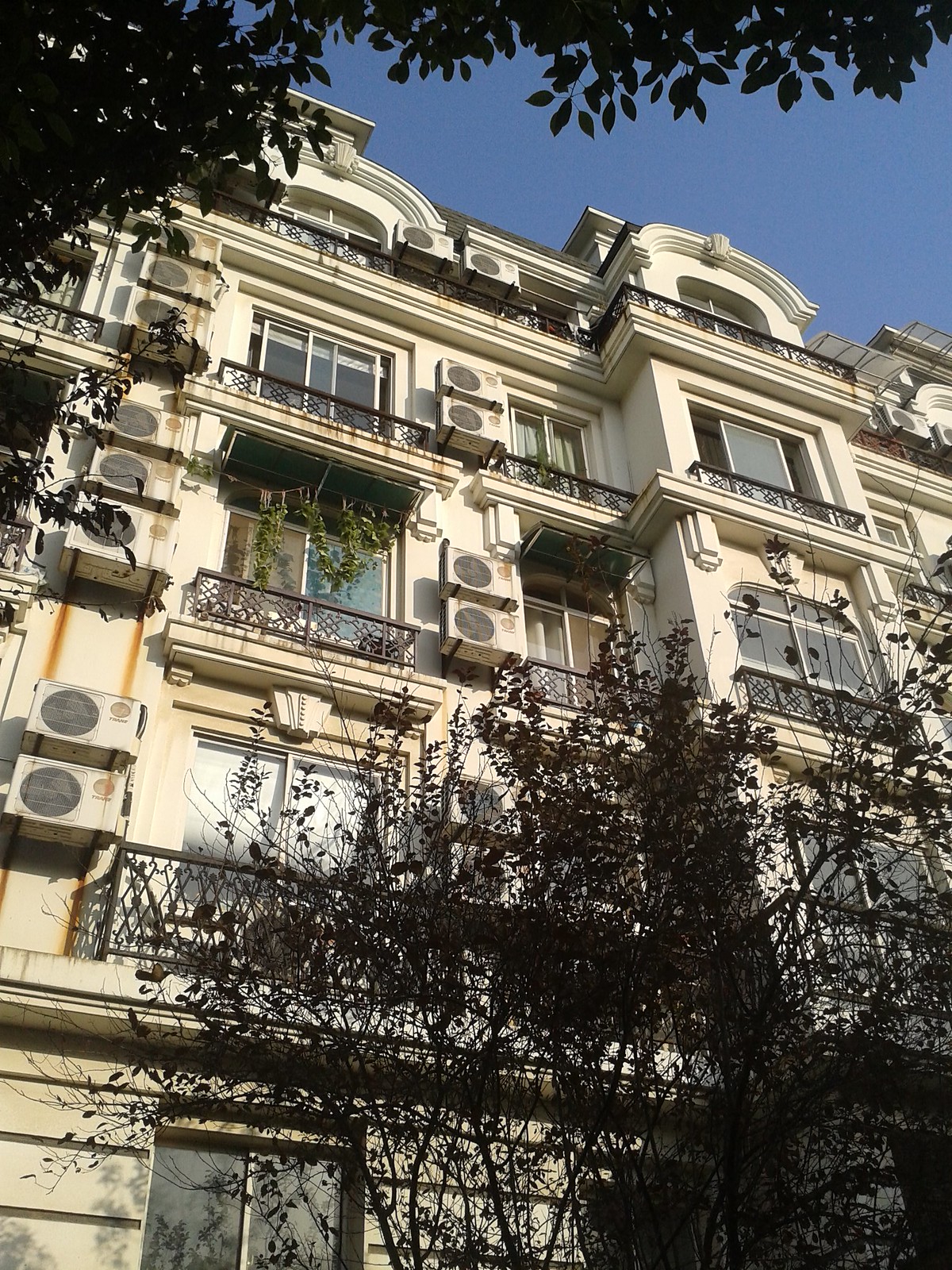This image depicts the exterior of a multi-story building, possibly a hotel or apartment complex, situated under a blue sky. The structure features five visible floors, each with continuous balconies adorned with black railings that incorporate diamond-shaped designs. The building's facade is white, with an ornate stone design and arches that lend a European architectural style. Numerous air conditioning units are strategically placed near the windows - specifically, two on the second floor, and three each on the third and fourth floors; the units on the fifth floor are obscured by tree branches. The balconies mostly house floor-length windows, and some have plants decorating them. The lower portion of the image shows trees with sparse, brown leaves, indicating they are not in the best health. The top floors appear to have larger balconies, suggesting possible penthouse units. Overall, the scene combines elements of residential and hotel architecture, captured in a clear and detailed outdoor setting.